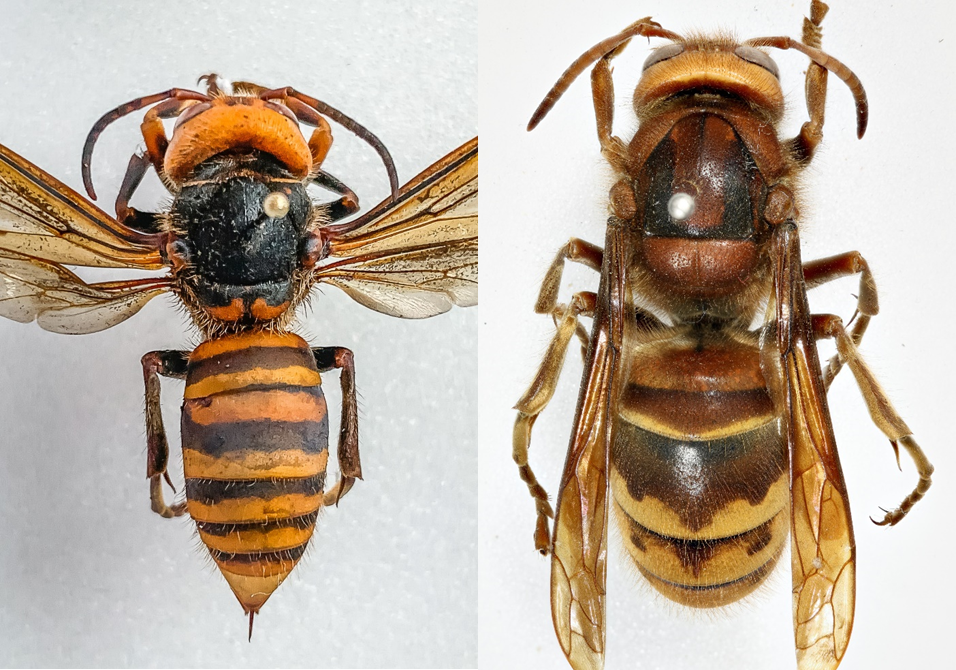This image features two side-by-side color photographs of bees, each pinned with a pearl-headed pin to a light gray background, arranged in a landscape orientation. The photograph on the left showcases a bee (or possibly a wasp) viewed from above. This insect has an orangish head with curled antennae, vibrant orangish-black eyes, and brownish pincers. Its body transitions from black between the head and tail to orangish and black horizontal stripes, with translucent, light brown-tinted wings outstretched. The bee's tail is pointed, extending behind a sharp needle.

The bee in the right photograph has a more rounded body shape with a golden-tan head, black eyes, and prominent antennae. Its body features a dark brown and beige-striped tail, with some minor dark brown patterning. The translucent wings, similar in color and form to those of the left bee, extend back on either side. Both bees are visibly dead, secured to their respective surfaces by pearl-headed pins through their central thoraxes. The overall style of the image is highly detailed and representational, focusing on the anatomical realism of the bees.